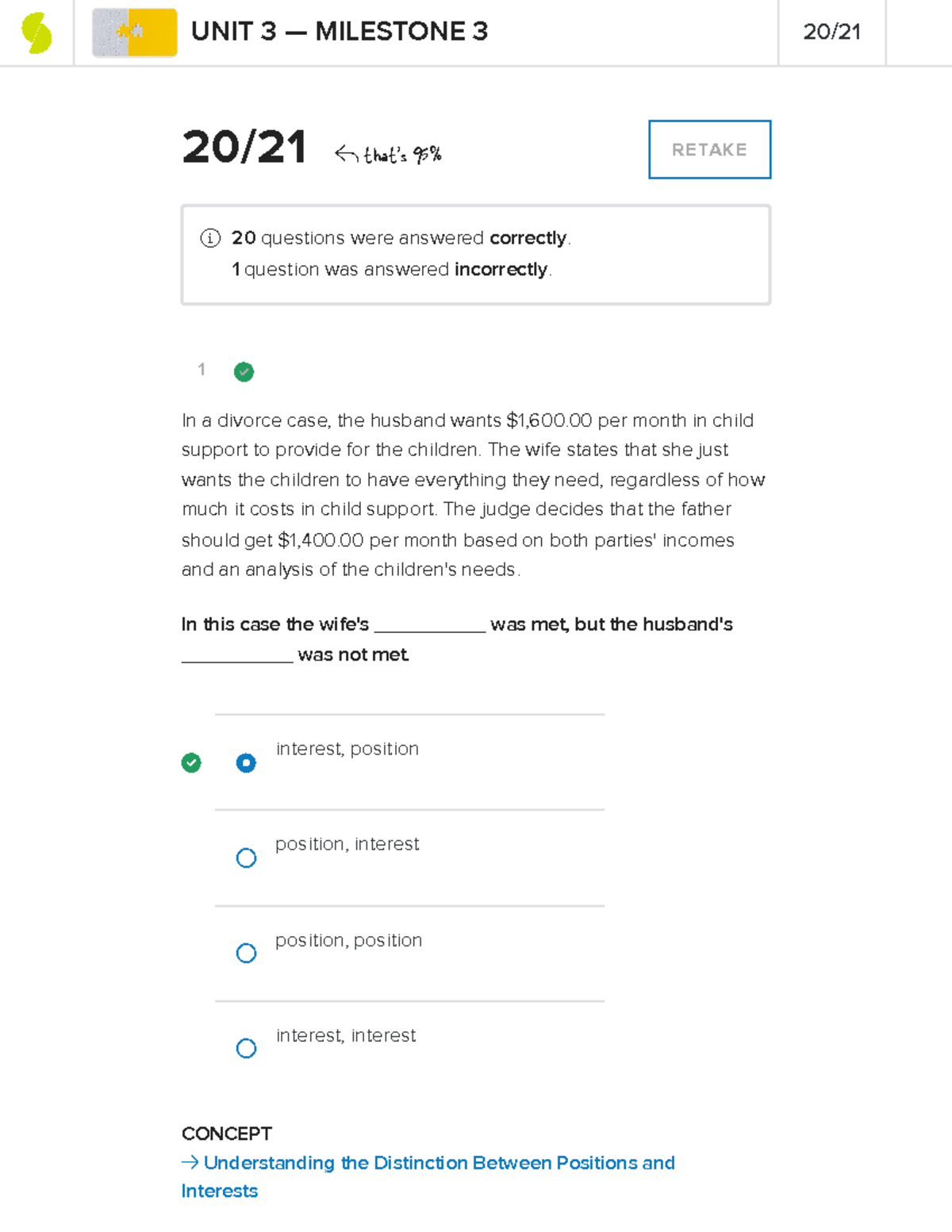The background of the image is predominantly white. In the upper left-hand corner, there is a half-cut green circle; part of the circle extends upwards while the other part slopes downwards. Adjacent to this is a thin gray vertical line. 

On the right side, occupying a substantial portion of the image and extending past the middle, is a mustard-colored rectangle. Next to it, a smaller section is gray. Within this gray section, in black text, it reads: "Unit Three - Milestone Three." Below this, there is a gray horizontal line followed by black text that reads: "20/21." Another gray line lies beneath it.

Further down, another horizontal gray line spans the width of the image. Below this line, there is black text reading: "20/21, 95%." 

Next to this, there is a box with a blue border, containing the gray text "Retake." Adjacent to it, another rectangle with a gray border contains black text stating: "20 questions answered correctly. One question was answered incorrectly." 

Below this, there is additional space followed by a green circle featuring a gray checkmark. Further down in black text is a scenario describing a divorce case: "In a divorce case, the husband wants $1,600 per month in child support to provide for the children. The wife states that she just wants the children to have everything they want, regardless of cost. The judge decides that the father should get $1,400 per month based on both parties' incomes and an analysis of the children's needs." 

Finally, the text concludes in black: "In this case, the wife's interest was met, but the husband's interest was not met." The scenario ends with a selection indicating "Interest position."